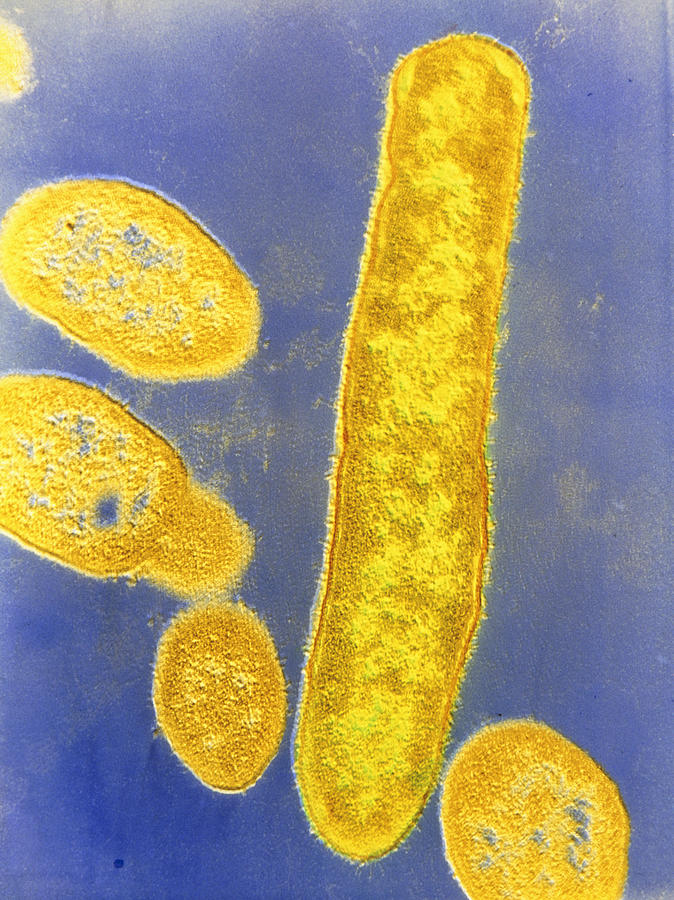The image showcases a vertically rectangular abstract artwork with a bluish purple background that features significant texture, suggesting the worn-off paint of a painting. The focal point of the piece consists of five distinct yellow shapes reminiscent of single-celled organisms, with part of a sixth visible in the upper left-hand corner. Most of these forms are oval or circular, containing hints of blue inside them, resembling microorganisms observed under a microscope. Notably, one elongated, worm-like shape on the right stands out with darker brown edges and fine hair-like structures, reminiscent of a stretched-out French baguette. The overall scene is dotted with yellow, contributing both to the dusty, powder-like texture and to the depth and intricacy of the composition.